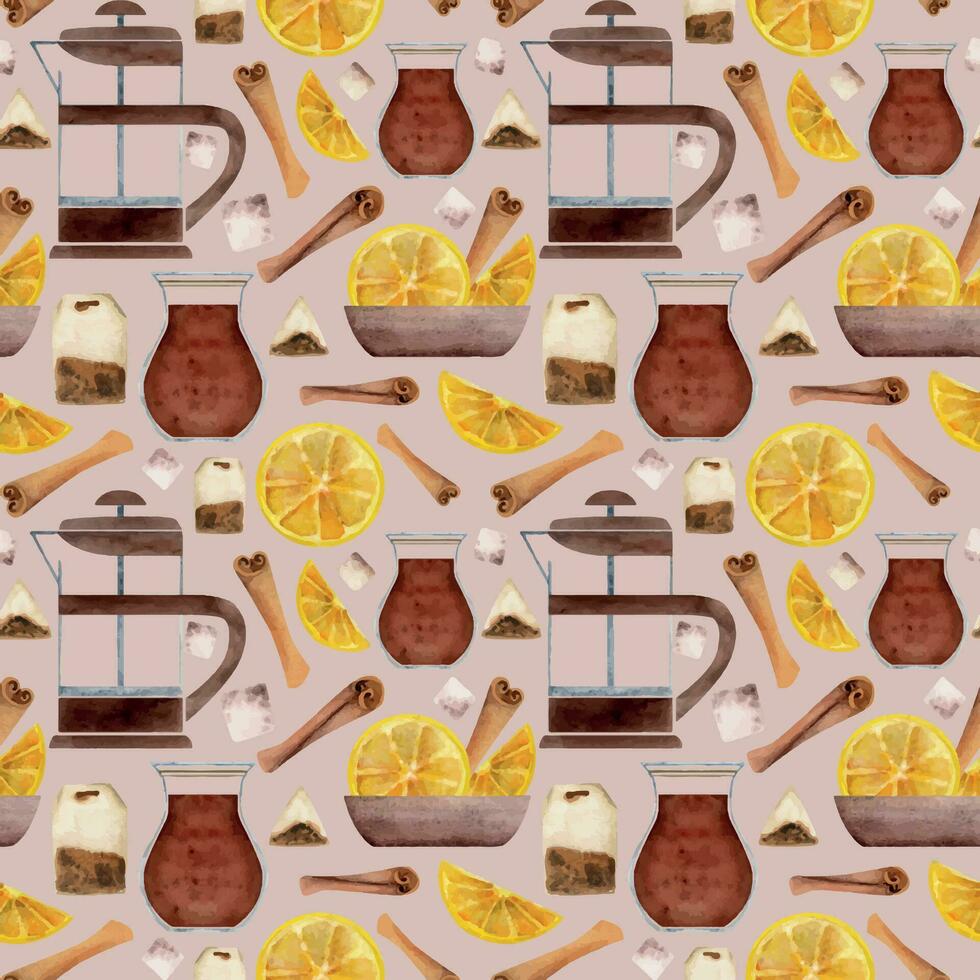This whimsical drawing, set against a light pinkish-gray background, features a repeated pattern of various tea and kitchen items. Dominant elements include four see-through kettles for brewing tea, filled with a brownish liquid that resembles iced tea, and eight identical pitchers, also likely containing iced tea. Scattered throughout are numerous slices and wedges of lemon, enhancing the citrusy theme, along with many cinnamon sticks, contributing a cozy, aromatic touch. Additionally, bowls containing a combination of lemon slices, lemon wedges, and cinnamon sticks are interspersed among the other items. The artwork predominantly showcases hues of yellow, brown, and maroon, creating a fun and engaging visual experience suitable for a kitchen poster.